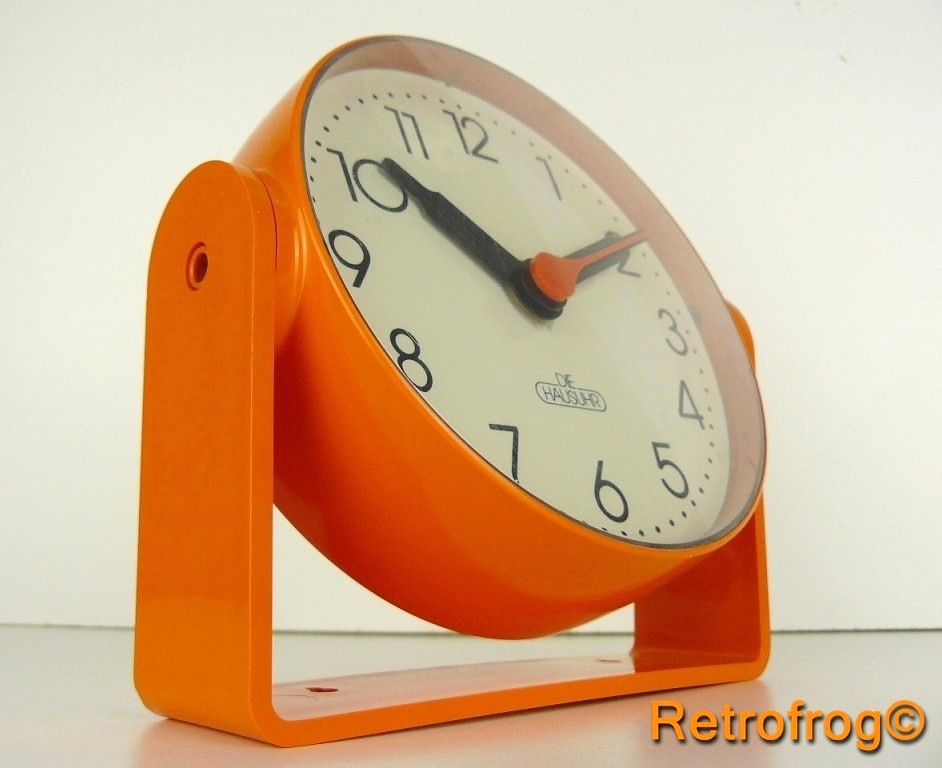The image features a vintage-style analog clock prominently positioned on a minimalist white surface, potentially a countertop or floor, against a plain white backdrop. The clock boasts a distinctive design with a flat cylindrical body reminiscent of a thick tuna can, dressed in a vibrant orange hue. Its round face is white with bold black hour and minute hands, accompanied by a striking orange second hand. The time displayed on the clock is approximately 2:51. Structurally, the clock is elevated and slightly angled upwards on a clear, U-shaped plastic stand, creating a contemporary aesthetic. In the bottom right corner of the image, the brand name "Retrofrog" appears in orange text, alongside a copyright symbol, suggesting either an advertisement or a professional photograph showcasing both product and branding.